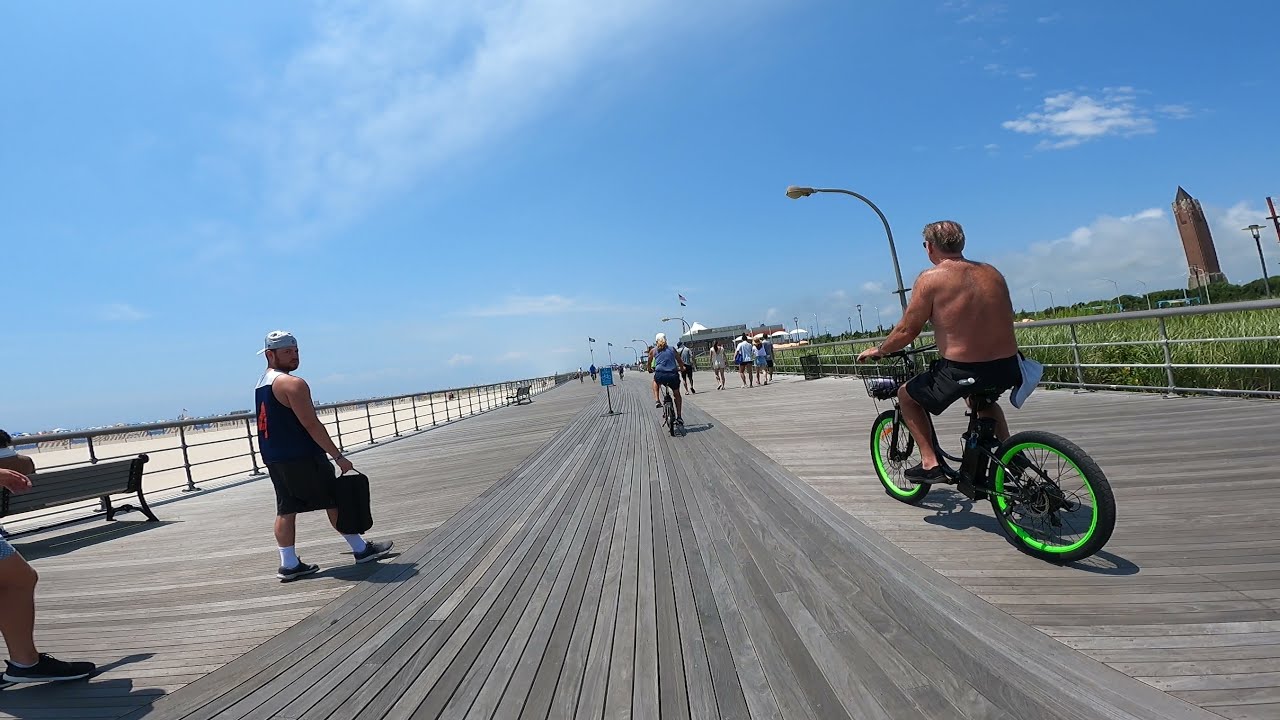The image is a vibrant color photograph of a bustling wooden beach boardwalk on a bright, sunny day with a expansive blue sky and a couple of white clouds. The scene centers around various individuals enjoying the boardwalk. To the right, an older shirtless Caucasian man rides a black bicycle with striking lime green rims, wearing black shorts and a white cap hanging from his waistband. Ahead of him, a woman is also biking. On the left side of the boardwalk, a man clad in a blue tank top, shorts, white socks pulled up to his calves, sneakers, and a backward white cap walks while holding a black tote bag, glancing back towards the camera. The boardwalk is flanked by a stretch of sand on the left, suggesting a nearby beach, although no water is visible. To the right, there is tall green grass, and far in the distance stands a large obelisk-like building resembling a brick version of the Washington Monument. Ahead, more people are seen walking and a few buildings can be spotted in the far background along with a bench and metal railing aligning the boardwalk. The photograph captures the lively atmosphere of a sunlit day at the beach boardwalk.